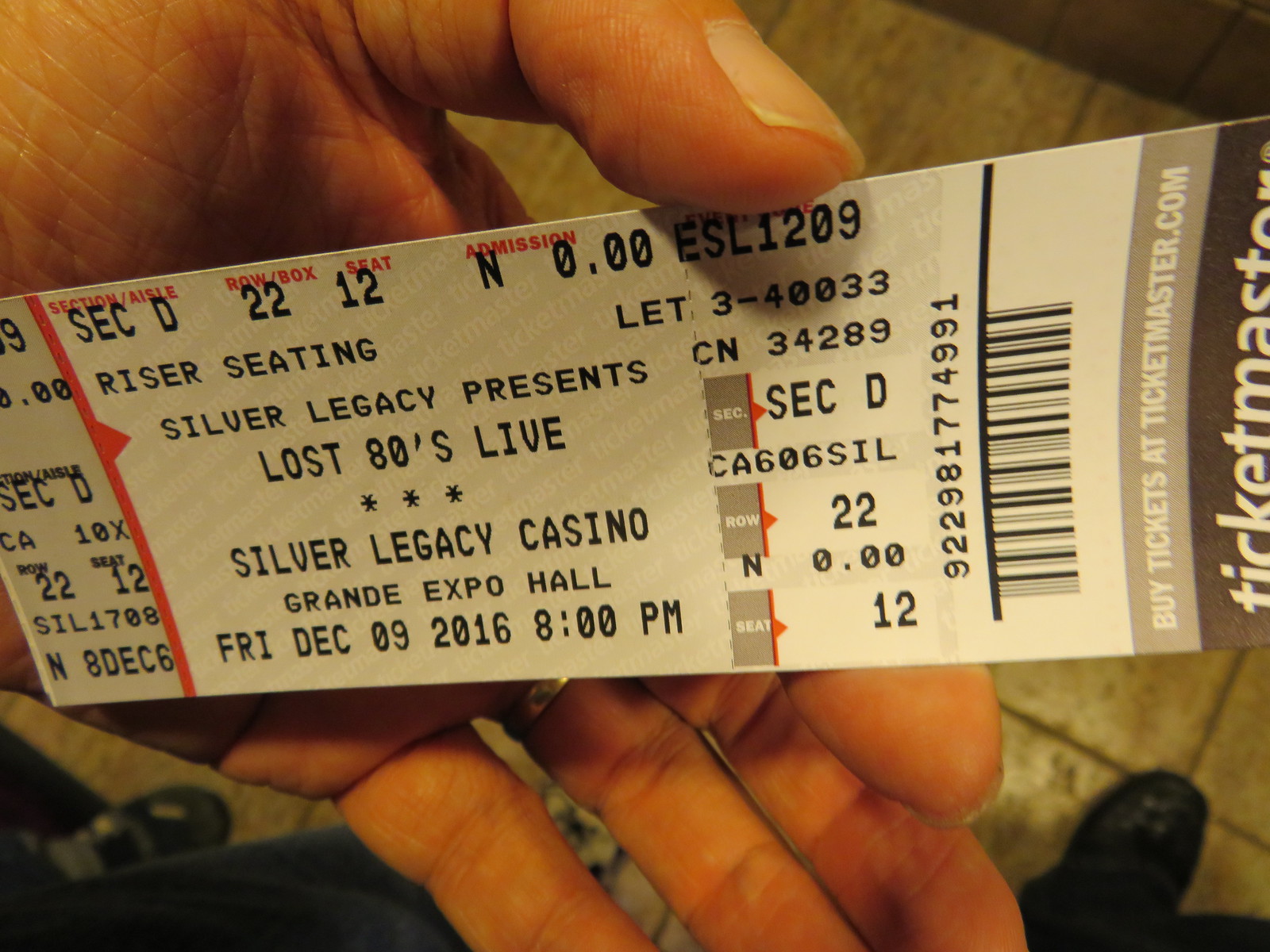The image is a close-up color photograph of a hand holding a concert ticket for the 'Silver Legacy Presents Lost 80s Live' event. The ticket is primarily gray with black text and some red markings. The detailed information on the ticket includes "Silver Legacy Casino, Grand Expo Hall, Friday, December 9th, 2016, at 8 PM." It specifies that the seating is in Section D, Row 22, Seat 12. The ticket features a barcode with the code 922-981-774-991, and there is also the familiar Ticketmaster logo along with an advertisement urging to "Buy tickets at Ticketmaster.com." The person's hand holding the ticket has visible fingernails and a golden ring. Beneath the hand, there's a tiled floor, and the shoes of this person, as well as another pair of shoes to the sides, suggest that two people are preparing for the event. The ticket is held in a palm-up position, pinched between the fingers and thumb, and the image captures the setting, seemingly indoors, around the time of the event in 2016.